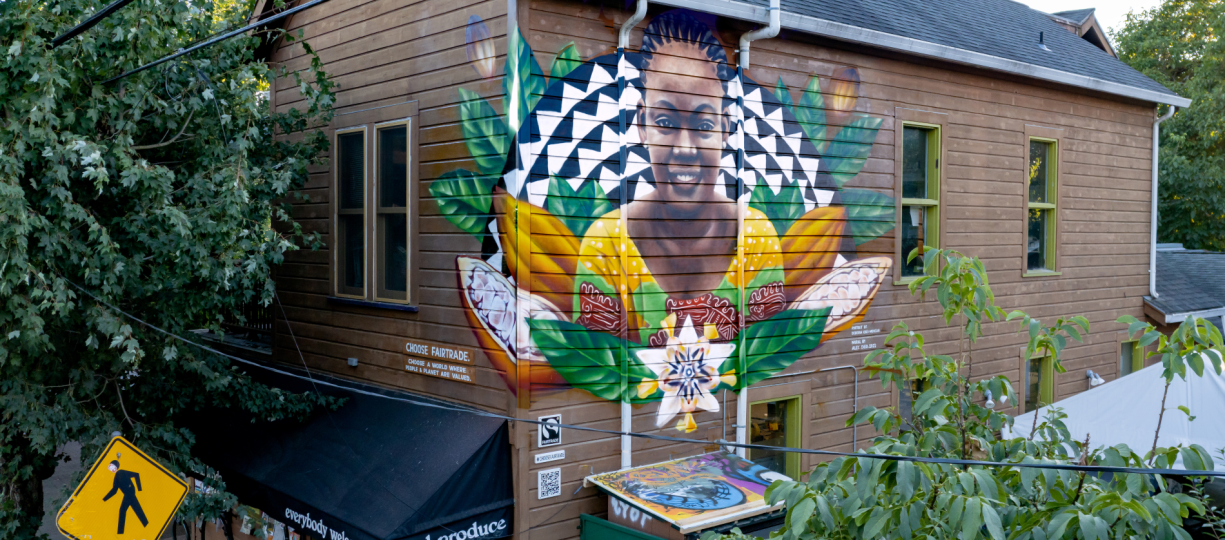The image depicts a wooden-sided building, possibly a house or a business, adorned with an elaborate mural of a woman with darker brown skin and black cornrowed hair. The woman, who could be African-American or Native American, wears a vibrant top in shades of yellow, green, and red. Surrounding her figure are lush green leaves and a semicircular rainbow pattern made of triangle shapes, along with white triangles on a black background. At the base of the mural, there are inscriptions like "everybody welcome," "produce," and "choose fair trade," along with a sign advocating for the value of people and the planet. The building features numerous windows, a black awning, and plants growing underneath the mural. To the left, there's a crosswalk sign in front of a tree, indicating a street nearby, and below the mural, partially visible, is a dumpster. The sun is low in the sky, adding to the detailed portrayal of this vibrant, community-oriented location.